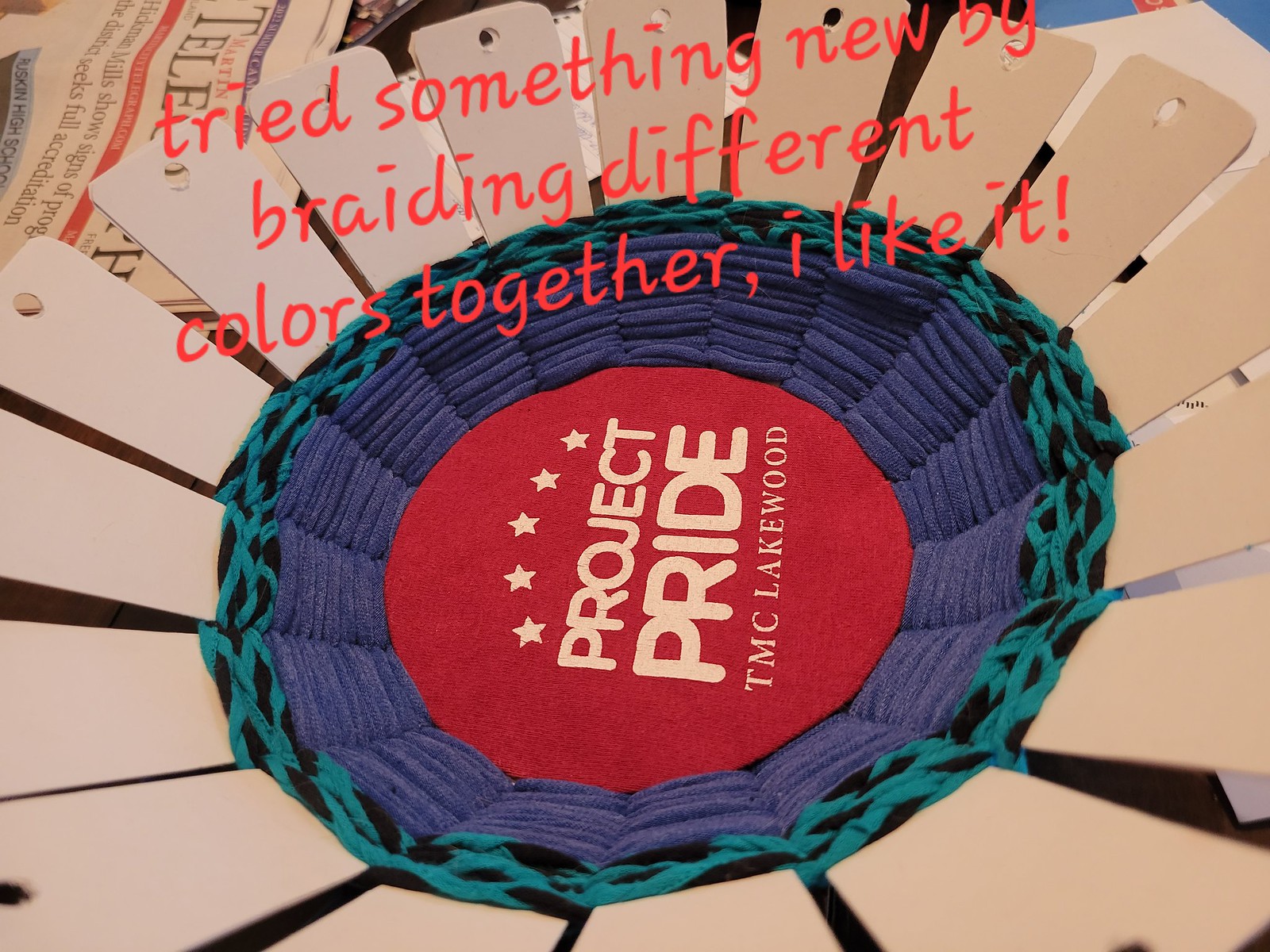The image is a detailed, wide rectangular photograph of a craft project centered around a circular red felt piece. This central felt circle features white, sideways text reading "Project Pride, TMC Lakewood," with five white stars forming a semicircle on the left side of the text. Surrounding the felt circle are multiple cardboard-like petals extending outward. Where these petals meet the felt, they are wrapped with various threads, notably dark blue and a turquoise and black pattern. Overlaying the image at the top, red text reads, "Tried something new by braiding different colors together. I like it." In the upper left corner of the image, there is a newspaper peeking into the frame. The entire assembly forms a bowl-like design with the cardboard petals angled upwards, and the background includes visible newspapers, books, and other crafting materials.